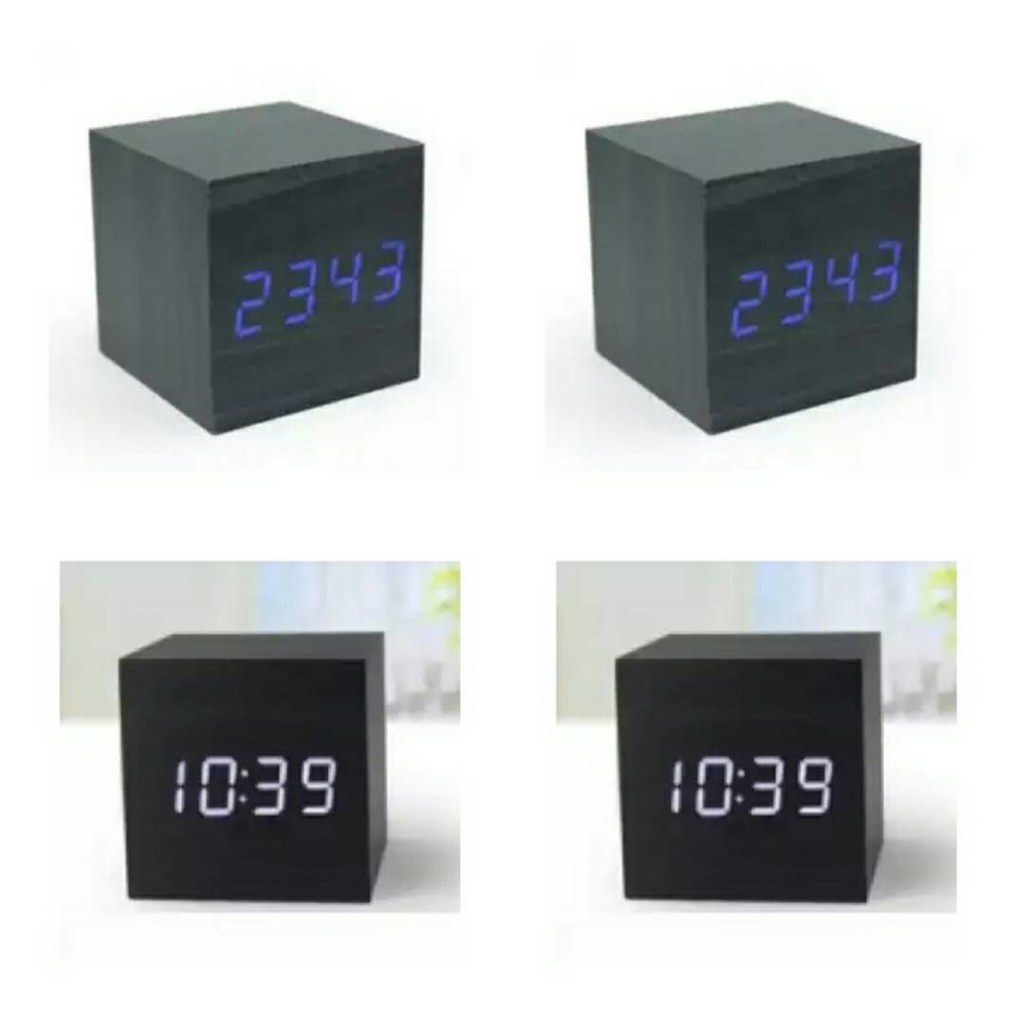In the image, we observe a collection of clock cubes. The top row features two identical gray cube clocks adorned with streaks of darker gray. These clocks display the time "23:43" in prominent purple digits. Beneath them, a second row showcases darker black cube clocks, which appear shinier and show the time "10:39" in illuminated numbers. Both sets of clocks are positioned on a white surface. In the background, a gray wall is partially covered by curtains. The curtains display a pattern with hues of blue, gray, and white, and a touch of yellow can be spotted on the right side. The overall composition captures a minimalist yet intriguing arrangement of timepieces against a subtly colorful backdrop.